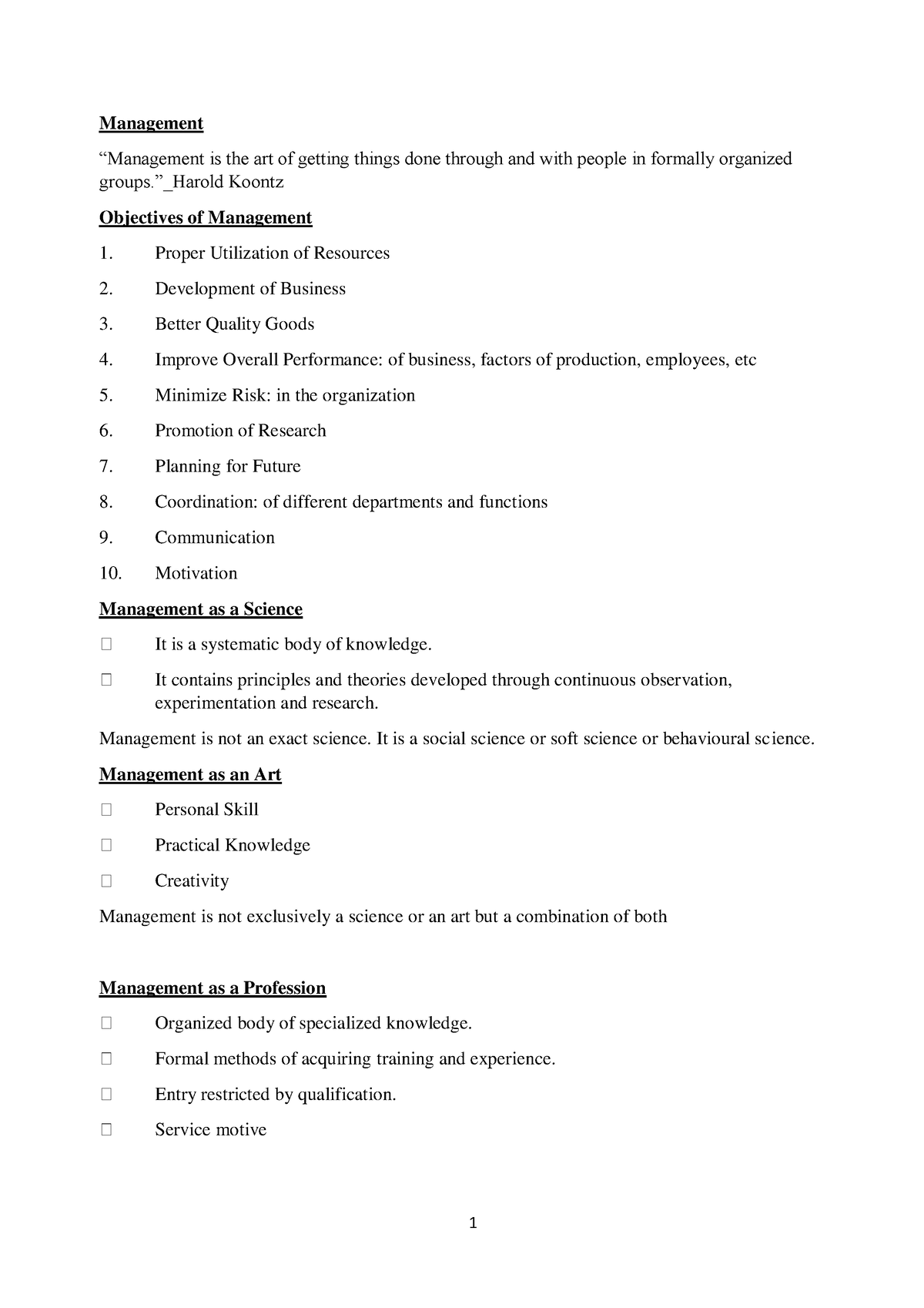The image displays a printed page featuring black type on a white background, with no specific indication of the originating location. The text on the page defines and elaborates on the concept of management, articulated through key points and bullet points. 

At the top, a quote by Harold Koontz emphasizes the definition of management: "Management is the art of getting things done through and with people in formally organized groups." 

Following this, the page outlines the **objectives of management** as follows:
1. Proper utilization of resources
2. Development of business
3. Production of better quality goods
4. Improvement of overall business performance, including factors of production and employee effectiveness
5. Risk minimization within the organization
6. Promotion of research
7. Planning for the future
8. Coordination of various departments and functions
9. Enhancement of communication
10. Motivation enhancement

The next section, underlined and titled "Management as a Science," presents the notion that management consists of:
- A systematic body of knowledge
- Principles and theories developed through continuous observation, experimentation, and research
  
It is noted that management is not an exact science but rather can be classified as a social, soft, or behavioral science.

The subsequent section discusses "Management as an Art," and highlights:
- Personal skills
- Practical knowledge
- Creativity
  
This section asserts that management integrates both scientific and artistic elements, forming a composite of both.

Finally, "Management as a Profession" is described with bullet points, recognizing it as:
- An organized body of specialized knowledge